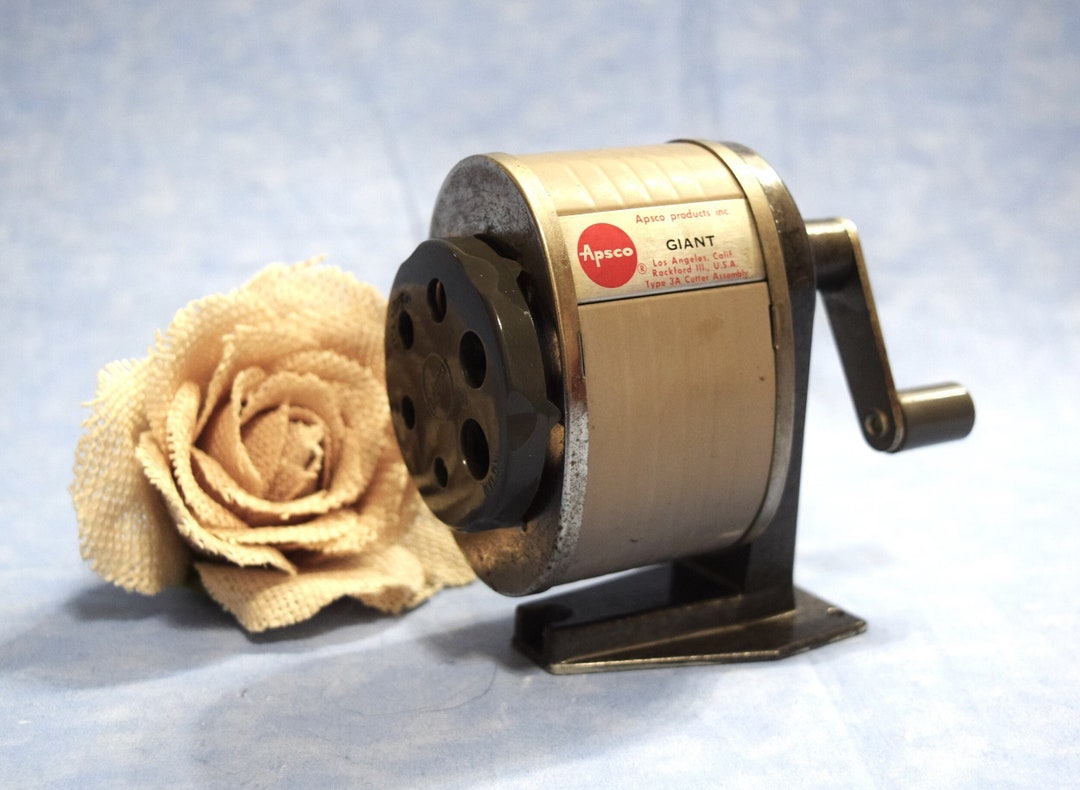This detailed image features a vintage, manual pencil sharpener marked by the brand name APSCO. Specifically, it is identified as the "Giant" model, indicated by embossed labels and a red circle with gold text that reads "APSCO." Additional labeling includes "APSCO Products Inc." in red, followed by "Giant" in black, and location information about Los Angeles, California, and Rockford, Illinois. The metal sharpener displays a blend of brown, tan, and copper hues. It is equipped with multiple openings of various sizes for sharpening pencils and includes a hand crank for manual operation. 

The pencil sharpener is set against a nondescript bluish-gray background, which is landscape-oriented, meaning the image's width is greater than its height. To the left of the sharpener, there is a cream-colored or beige artificial flower that resembles a rose. The flower appears to be crafted from felt or a similarly textured fabric. There is no defined pattern in the background, lending the scene a subtle and muted aesthetic.